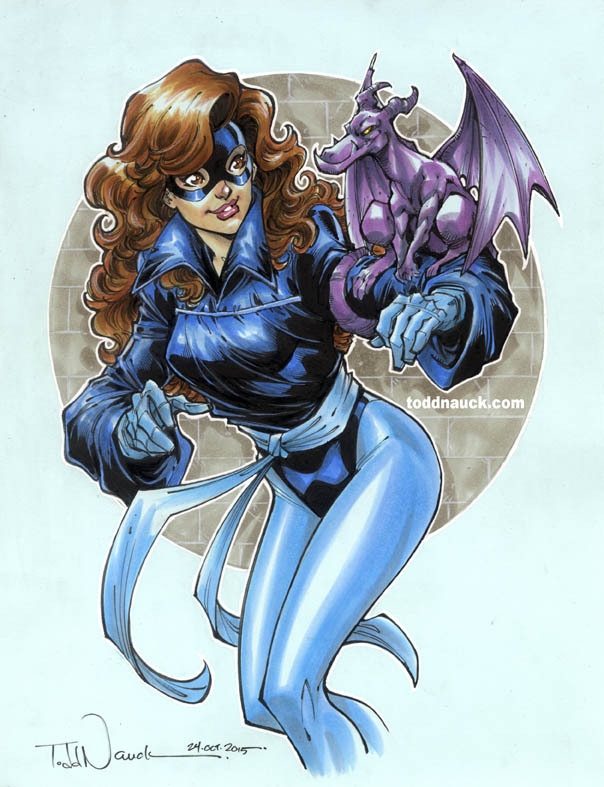The image is an artist's drawing of a young woman who appears to be a superhero, set against a light blue or light bluish-green background. She has long, dark brown, shiny curly hair and is dressed in a uniquely designed blue outfit. The outfit consists of a slightly baggy top with a large blue collar, shiny light blue tights, and a blue belt tied at the waist, hanging down. Her hands are clad in blue gloves, and she wears a dark blue mask over her eyes and forehead, similar to the style of Robin from Batman and Robin, but allowing her expressive eyes and red lips to be visible.

Perched confidently on her extended left arm is a small purple dragon with yellow eyes and tusks protruding from its upper jaw, its wings slightly extended as it sits smugly. The background behind her features a circular design with a gray brick pattern that frames her figure from the head to the middle of her legs.

At the bottom right of the image, the text "ToddNAUCK.com" is present, indicating the artist's name and website, with the date "24 October 2015" possibly noted as part of the artwork.